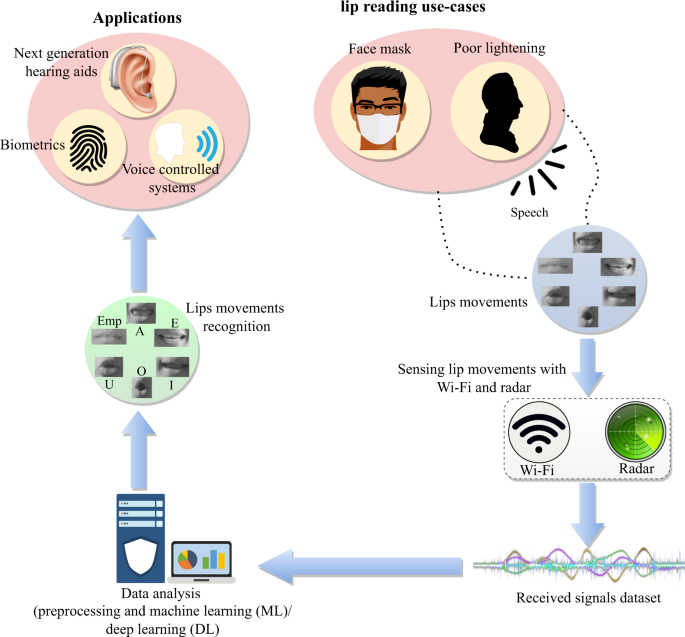The diagram appears to depict the process and use cases of advancing lip reading technology. At the top right, it is labeled "Lip Reading Use Cases." The diagram features a sequence of images and text, connected by arrows forming a flow from the upper right, looping downwards to the bottom left, and back up towards the right. 

In the upper right corner, there's a pink oval showing a person wearing a face mask alongside a dark image representing poor lighting conditions, indicating scenarios where traditional lip reading is challenging. Arrows lead to the next stage, which features close-up images of lips in motion labeled as "lip movement." Following these, the process showcases the use of Wi-Fi and radar technologies to sense lip movements, indicated by respective icons.

Next, an arrow points to a section labeled "Receiving Signals Dataset," from which another arrow directs to "Data Analysis." Here, terms like Preprocessing, Machine Learning, and Deep Learning are noted. Subsequently, the diagram shows this processed data moving back to another set of lip images, reinforcing the recognition aspect.

Finally, the arrows lead to the top left corner, titled "Application." Illustrations of an ear, a fingerprint, and a person speaking are accompanied by text listing the potential applications: "Next-Generation Hearing Aids," "Biometrics," and "Voice-Controlled Systems." Overall, the diagram comprehensively illustrates the pathway from initial sensing of lip movements in challenging conditions to potential advanced technological applications.